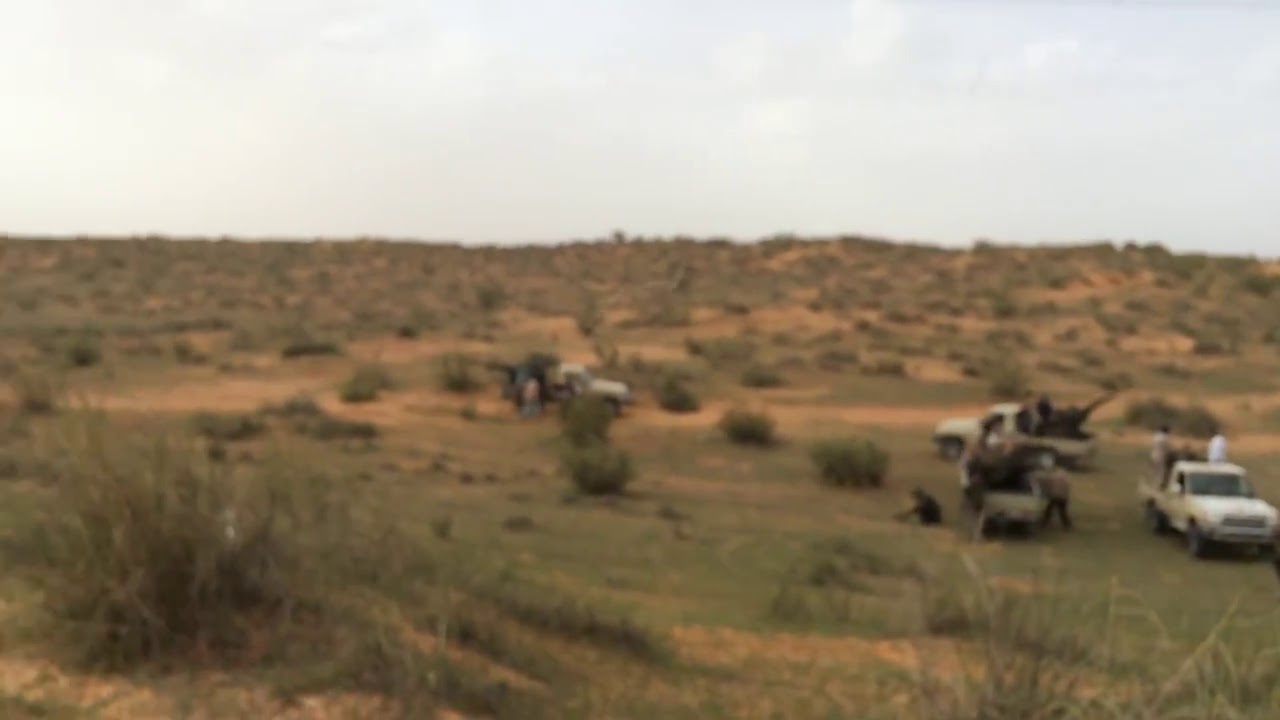This photograph captures a mid-day scene in a desolate, grassy, and somewhat hilly field. The landscape features sparse and patchy vegetation, with green grass, weeds, and patches of brownish-beige dirt. Located predominantly in the bottom right and center of the image are several small pickup trucks, which appear beige or white. Most of these trucks have trunks or beds filled with men, although the image is blurry and the details of these individuals are difficult to discern. The men are seen standing around the vehicles, and there are suggestions of possible military presence with mentions of guns and long, arm-like structures in the trucks' beds, potentially hoists. The sky above shows a light blue hue with faint white clouds, indicating clear weather. This combined setup suggests a possible outdoor gathering, perhaps for a safari, militia, or sightseeing in this wide-open, arid area.